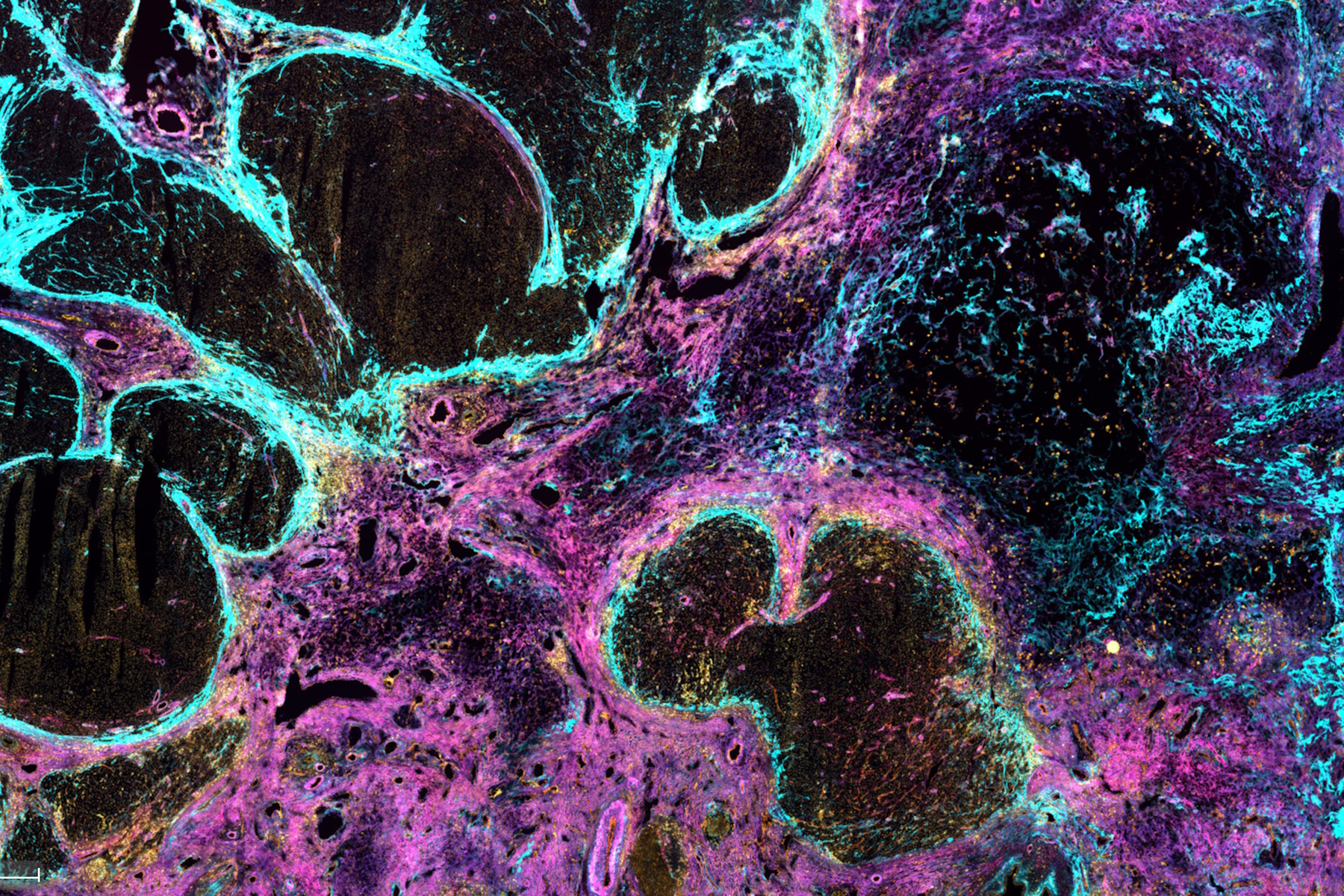The image is an abstract composition featuring a variety of circular and oval shapes set against a predominantly black background, resembling a chalkboard. The colors are vivid and diverse, with prominent shades including dark brown, black, teal, various purples, mauve, pink, light pink, fluorescent green, and orange. These neon-like colors create a dynamic and vibrant visual experience. The shapes, which appear spongy and reminiscent of cells or bacteria under a microscope, lend a textured and organic feel to the image. The larger shapes are mainly teal and purple, often surrounded by blue, with smaller orange and pink dots scattered around. This creates a sense of motion or activity, as if the elements are moving or interacting. The black background effectively contrasts and offsets the bright, lively colors. Overall, the image has no discernible objects, borders, or text, focusing purely on the interplay of shapes and colors to evoke an abstract, almost microscopic view.